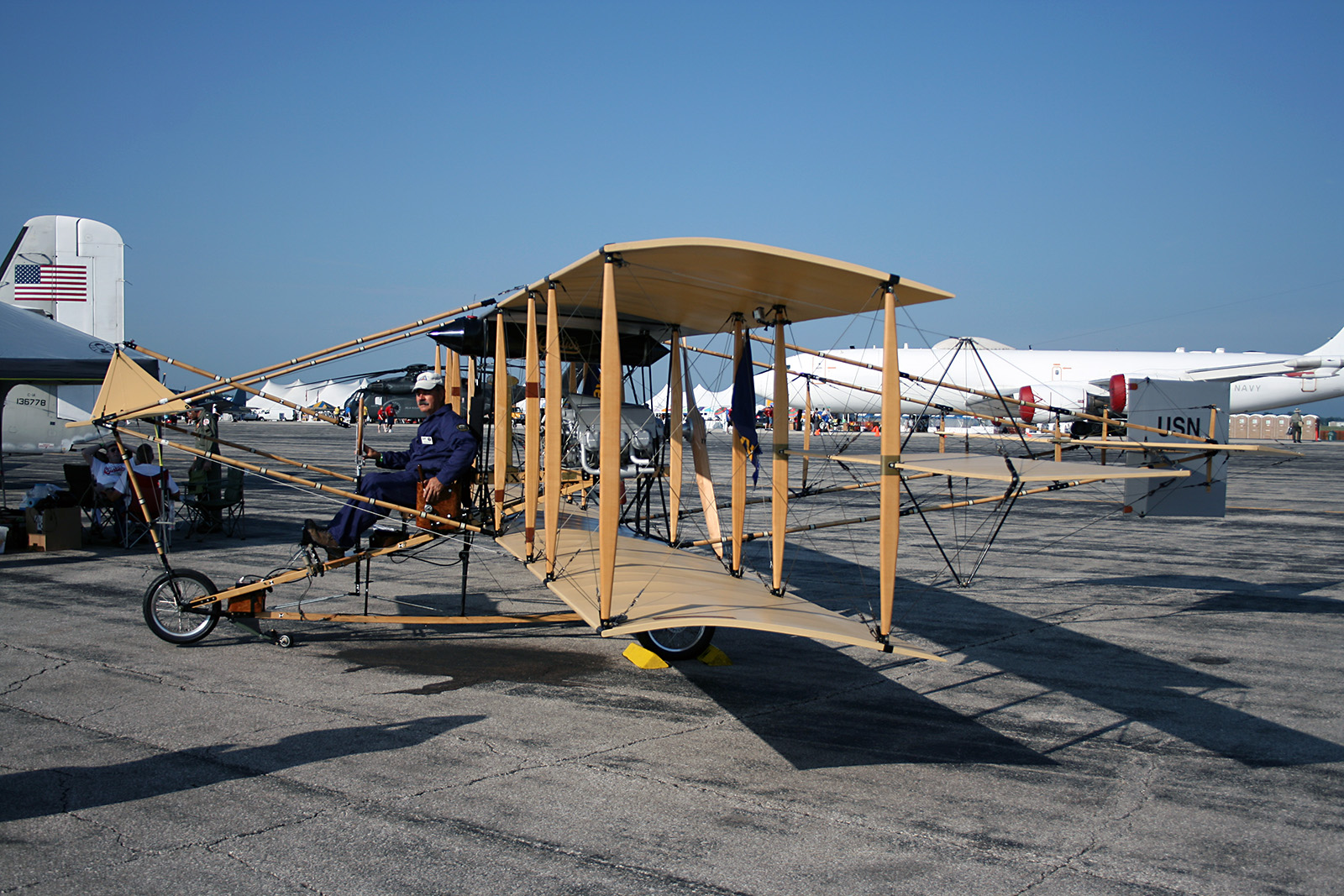The photo captures a striking scene at an airfield, possibly resembling Denver International Airport due to visible white canopies. Dominating the foreground is an old-style biplane reminiscent of the Wright brothers' design, featuring two wheels at the bottom and multiple rows of wings held together by wooden columns and tensioned strings. Despite its vintage appearance, the aircraft looks fairly new, likely a modern reconstruction. Seated in the cockpit is a man wearing a blue outfit and a white hat, looking directly at the camera. The biplane rests on a concrete runway amidst several modern commercial planes, identifiable by their sleek, white structures. The blue sky provides a clear backdrop, and toward the right-middle of the picture, a group of people gathers under a tent. Notably, there is an American flag visible on the wing of another aircraft to the left-middle, adding a patriotic touch to the scene.